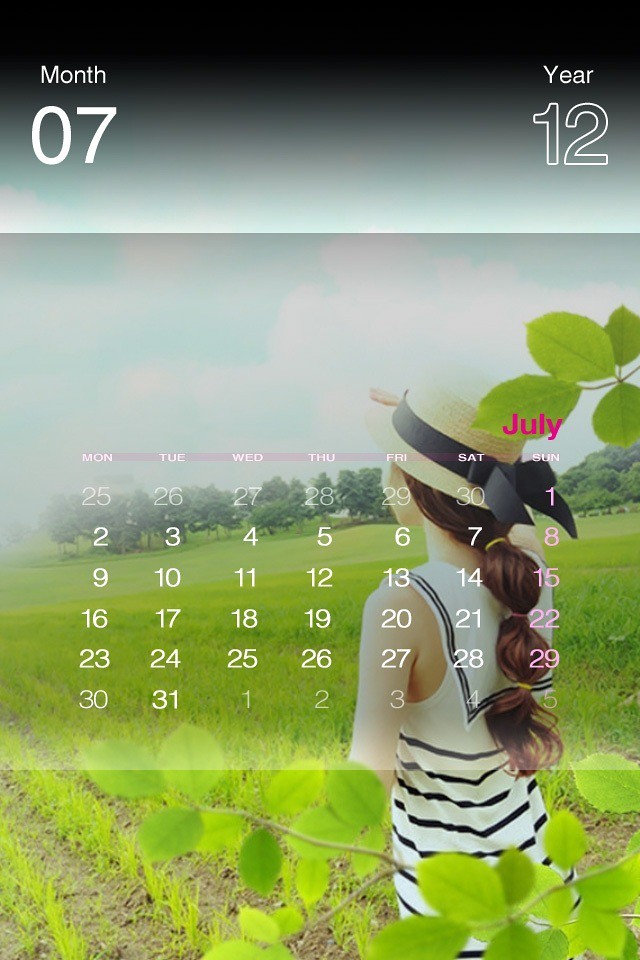The image is a vertical screenshot of a calendar taken from a mobile device. At the top, there's a black banner with white text displaying "month 07, year 12." Below this banner, the main calendar occupies the majority of the screen, with a grid layout featuring seven columns and seven rows. The days of the week are abbreviated to three characters (Mon, Tue, Wed, Thu, Fri, Sat, Sun) and the dates span from the 25th of the previous month to the 5th of the next, with a notable pink highlight indicating "July." The calendar has a grey background, with the day numbers and weekday names in white text.

Behind the calendar, the background shows a scenic farm setting. There is a blue sky with white clouds at the top, and green trees and leaves scattered throughout the image. The ground has a mix of green grass, brown dirt patches, and some yellowing areas. A girl stands in the field wearing a beige summer hat with a black band, a black and white dress, and her hair tied back. Her pose suggests a casual stance—one hand above her head and the other by her side. Overall, this image captures a serene farm landscape with a prominently featured mobile calendar interface.